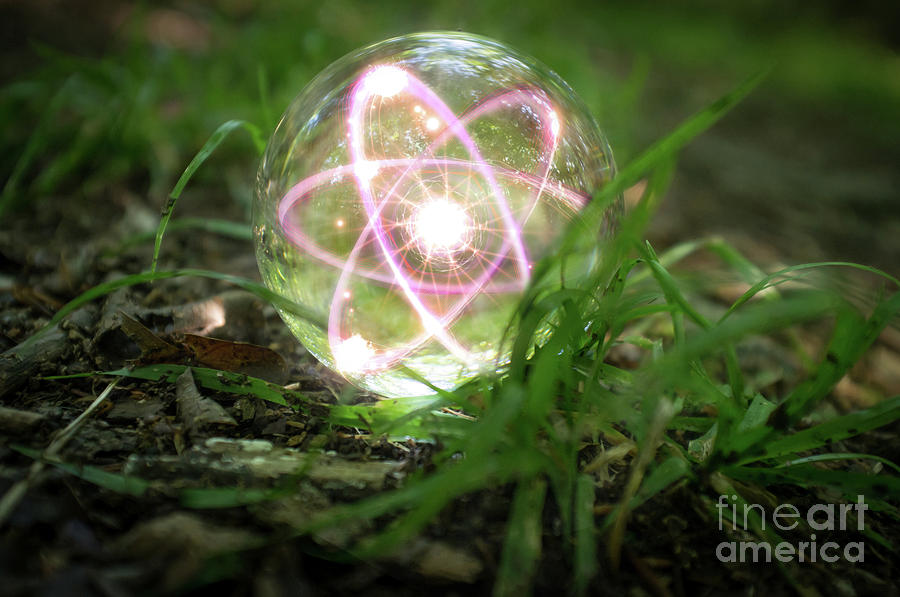The digital artwork presents a photorealistic nature scene featuring a lush green ground with grass, brown leaf debris, twigs, and branches. At the center of this earthy setting lies a translucent, reflective glass sphere, akin to a water bubble. Inside this sphere is an atom-like structure, glowing with an ethereal pink and white energy. The nucleus of this atomic structure emits light beams, with fibers extending towards three distinct ovals, which form rotating, energy rings arranged diagonally to the top left and right, and one horizontally, enhancing the impression of an atomic symbol. The background showcases a bokeh effect, adding to the artwork's mystical ambiance. In the bottom right corner, a watermark in faded white lowercase text reads “fine art america,” with "art" and "america" in bold. The glass sphere serves as the primary light source, illuminating the otherwise dimly lit scene.